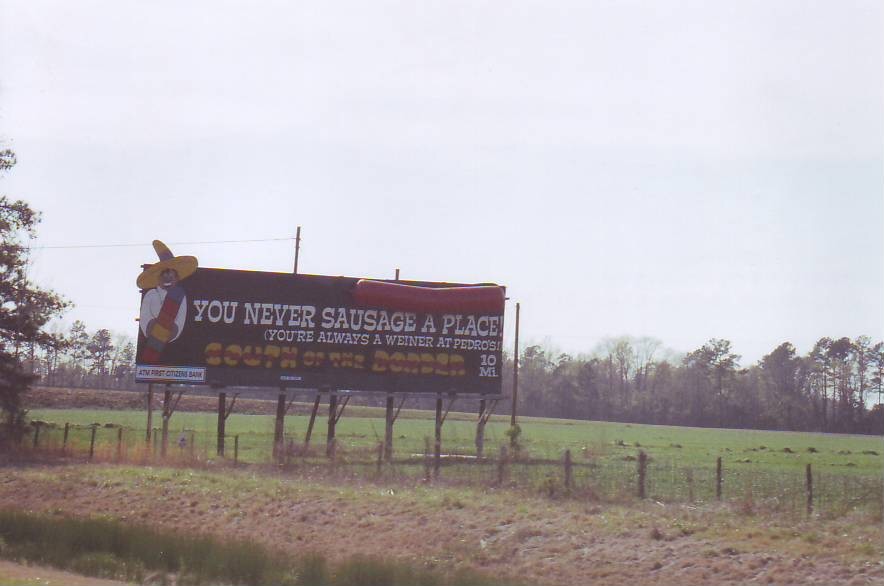This color photograph captures a rural roadside scene dominated by a vibrant, eye-catching billboard situated in a grassy field. The photograph is taken from a slightly angled perspective, emphasizing the rustic foreground, complete with green grass, fence posts with wire fencing, and a dry slope dipping into a ditch. In the distance, a horizon filled with trees frames the billboard, and the sky above is overcast with gray clouds.

The billboard itself stands out due to its dark blue or black background and vivid illustrations. On its left side is a caricature of a man with dark skin, wearing a large, yellow sombrero and a white shirt, along with a colorful scarf that drapes over his left shoulder. The sign's text catches the eye; the top line reads "You never sausage a place!" in bold white letters, directly below it in slightly smaller white text is, "You're always a wiener at Pedro's!" Flanking the upper right corner is a striking three-dimensional sculpture of a sausage that curves slightly downward in the middle, projecting out from the billboard. Below the main text, a stylized tagline "South of the Border" is displayed in a playful bubble font with undulating red and yellow colors, resembling ketchup and mustard, perhaps over a hot dog bun. A final line marking the distance to the location, "10 miles," is also noticeable.

The composition of the photograph and the vivid details of the advertisement make it a striking image, blending humorous text with dynamic visual elements against the subdued backdrop of the countryside.